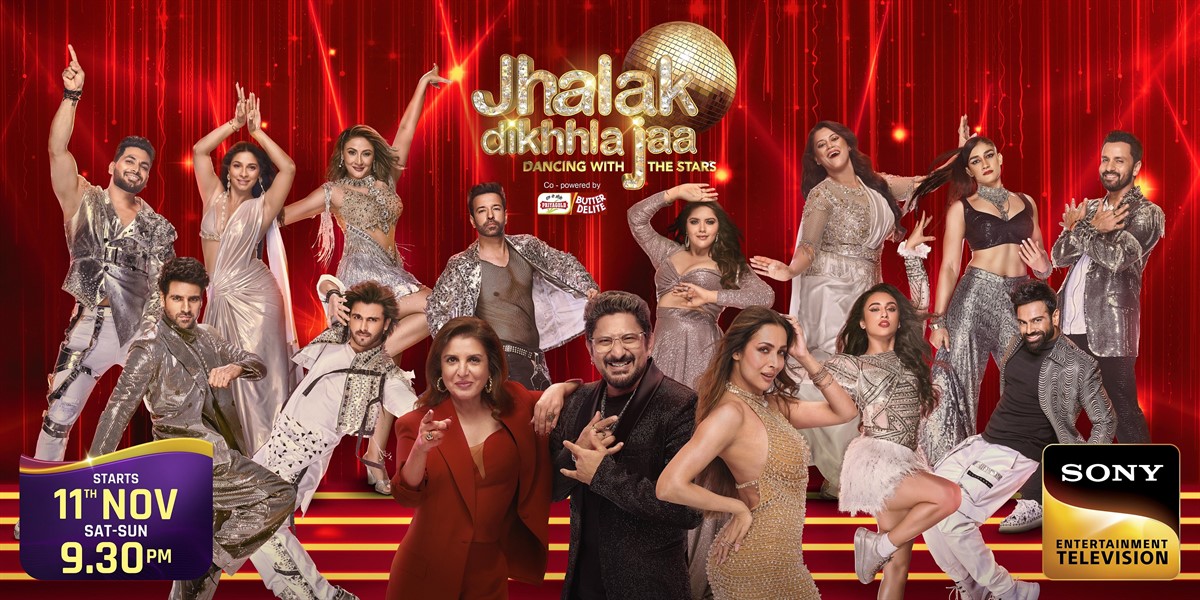The image is a vibrant advertisement for "Jalak Dikla Ja," an Indian adaptation of "Dancing with the Stars." The poster features a captivating array of dancers dressed in shimmering silver outfits, posed elegantly in front of a rich red curtain, with a sparkling disco ball hanging at the center. Prominently in the foreground are the show’s hosts: a middle-aged woman in a striking red pantsuit, a middle-aged man in a sleek black suit wearing glasses, and a woman in a stylish, slinky gold-beaded dress posing sassily. The poster includes crucial details in the lower left corner, highlighting that the show airs from 11th November, Saturday through Sunday, at 9:30 PM. On the right side is the logo for Sony Entertainment Television. The background is filled with images of 12 dancers, each striking dynamic dance poses, showcasing their enthusiasm and energy for the upcoming competition.